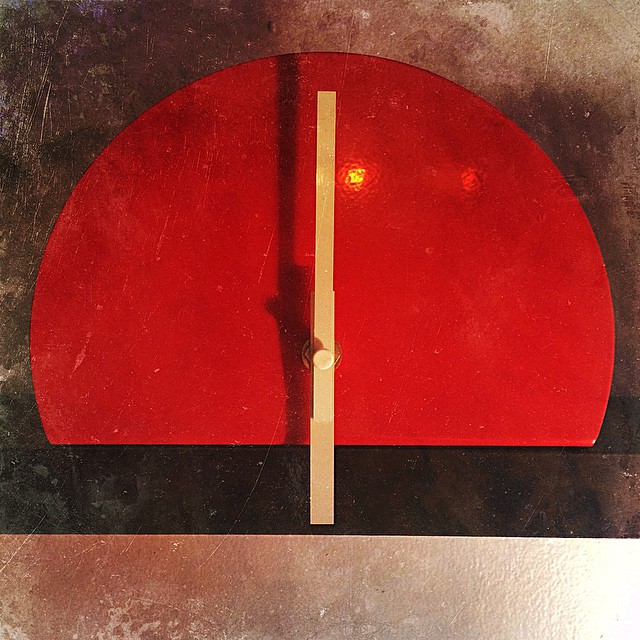The image depicted appears to be a vintage elevator floor indicator set against a background that resembles polished stone. The background predominantly displays a glossy brown surface, transitioning to a more peachy hue in the upper right corner. Central to the image is a red, semi-circular dial—approximately two-thirds of a complete circle—with a small, gleaming yellow reflection on its surface. Below the dial, a tan-colored wooden arm points upwards, casting a shadow behind it. The absence of numerical indicators on the dial suggests an old-fashioned design reminiscent of classic elevator displays, where the arrow would traditionally move to indicate the current floor.